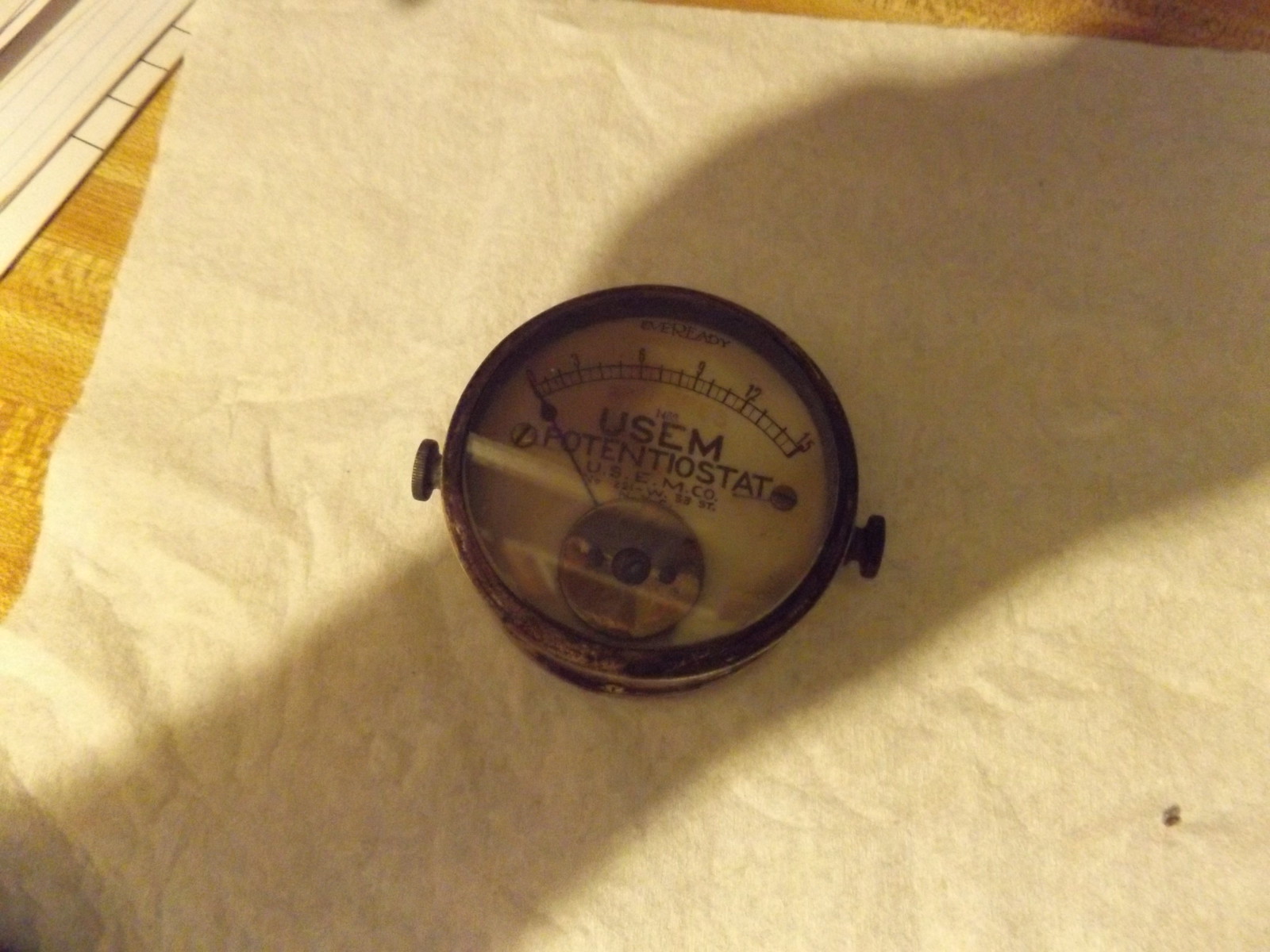This image showcases a vintage potentiostat, specifically a model from the USEM Company. The device is positioned atop a substrate that appears to be either a piece of cream-colored felt or paper, which is placed on a wooden counter or tabletop. Surrounding the potentiostat, particularly in the upper left corner, are scattered papers.

The potentiostat features a white-faced gauge encased in a metal housing with a clear glass cover. The words "EverReady" are prominently displayed at the top of the gauge. The dial, which has a single indicator hand, is marked with numbers ranging from 0 to 15 in increments of 3, with the numerical and textual details printed in black.

On either side of the gauge are two knobs, whose precise functions are unclear, but they might be designed to secure the meter in place or possibly serve as rotation controls. The face of the gauge also includes two visible screws. This intricate detail provides a glimpse into the careful craftsmanship and enduring design of this historical instrument.